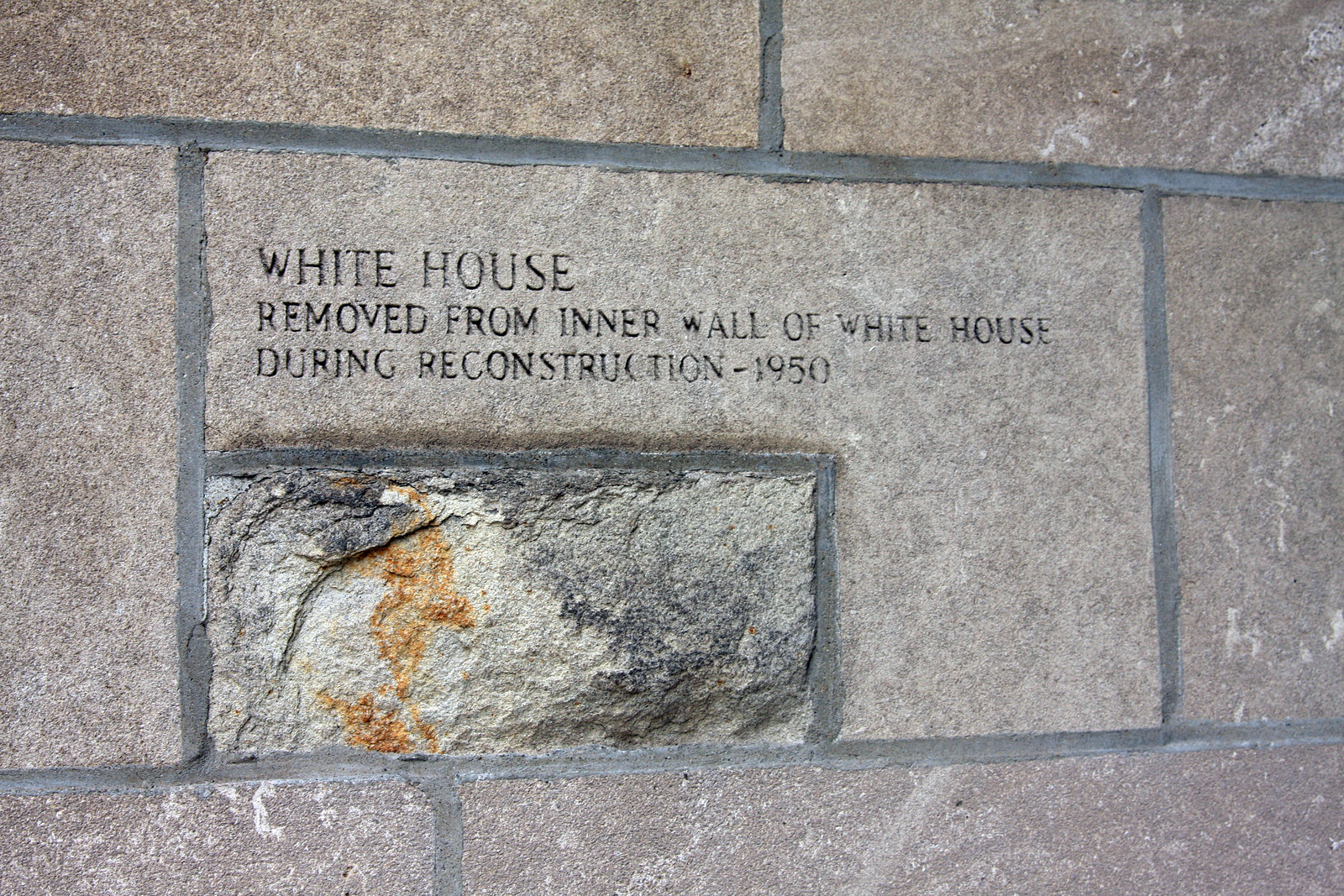The image depicts a brick wall with prominent white grout between the bricks, set outdoors in daylight. At the center of the image, there is a large, jagged brick with black and orange stains, distinguishable from the smoother, more uniform-colored surrounding bricks. This central brick features an engraving that reads: "White House, removed from inner wall of White House during reconstruction, 1950." Just below this engraved brick, inset into the wall, is a smaller brick. The overall color palette of the image includes shades of brown, white, gray, black, and orange.